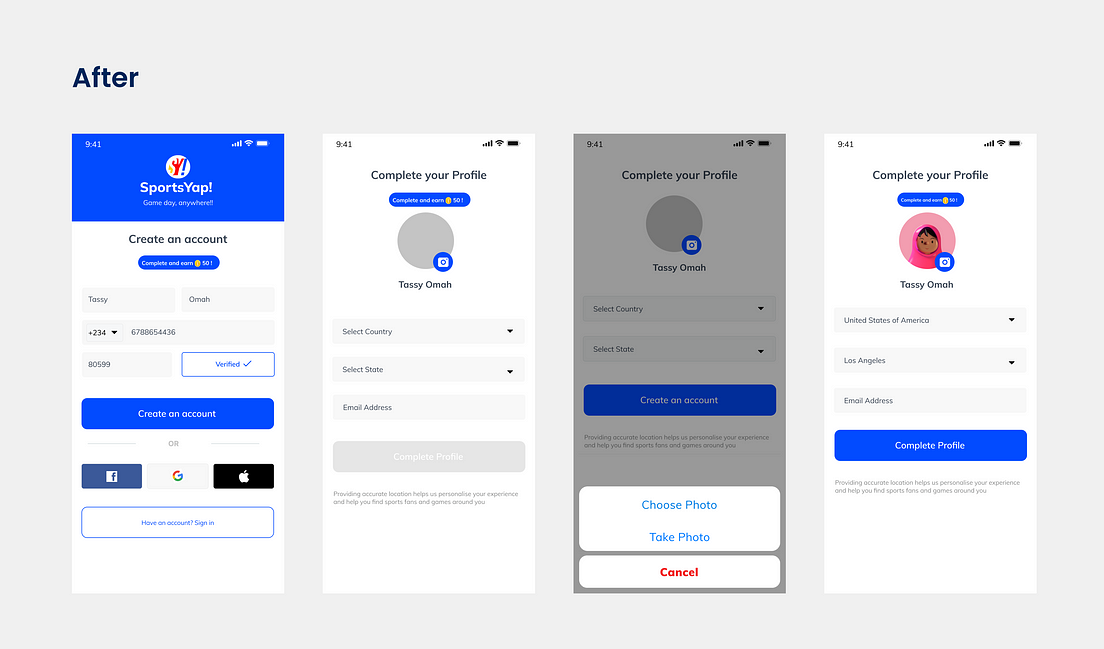The image portrays a composite of four side-by-side mobile phone screenshots set against a solid light gray background. In the upper left-hand corner, bold black text reads "After." Below that text is the first screenshot showcasing the "SportsYap" app. This screenshot features a blue banner with "SportsYap" written on it. Beneath the blue banner, it has a white background with "Create an Account" in black text. There is a visible blue button and several input fields for first name, last name, phone number, etc., followed by verification prompts. An option to sign in with Facebook, Google, or Apple accounts is also displayed.

The second screenshot focuses on completing the user profile, illustrating additional input fields for more personal information.

The third screenshot guides the user on how to upload a profile photo, detailing the steps needed for this task.

The fourth and final screenshot revisits the "Complete Your Profile" page from the second screenshot, now updated to include the user's newly uploaded profile picture.